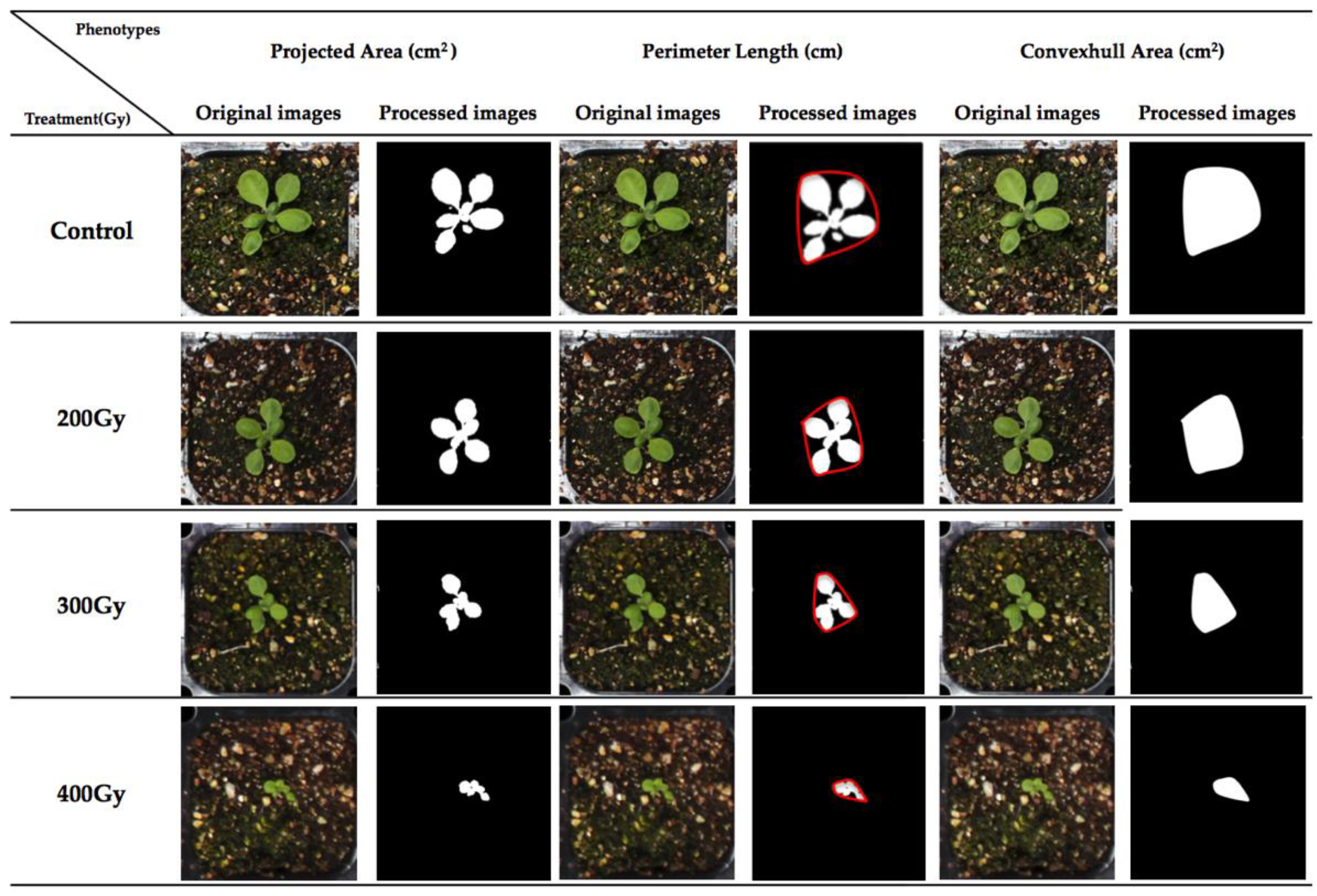This image shows a detailed study of plant growth under various treatments, as presented in a textbook. The collection is arranged in a grid pattern, with four rows and six columns. Each row represents different treatments labeled as control, 200 GY, 300 GY, and 400 GY down the left side. The columns across the top are labeled progressively with projected area (cm²), perimeter length (cm), and convex hull area (cm²) for both the original and processed images. Each cell in the grid contains paired images. The original images, situated in the first of the paired columns, are close-up views showing a green, young plant with about six leaves against the soil. The processed images, situated in the second of the paired columns, display a black background with the white contour of the plant’s processed area. As the treatment intensity increases from control to 400 GY, the images demonstrate a noticeable decline in plant health.